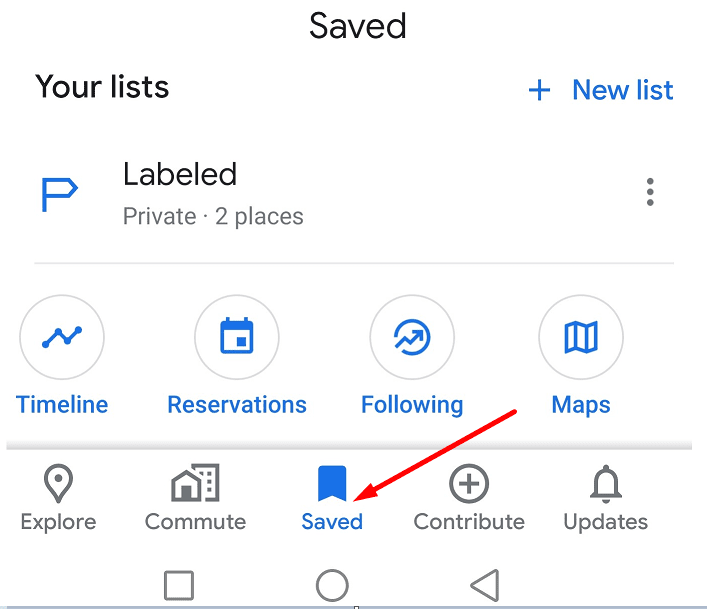The image showcases a section of a website interface. At the very top, the word "Saved" is displayed prominently in black text. 

On the left side of the screen, a menu item labeled "Your Lists" can be seen, while on the right side, there is a blue button labeled "New List" accompanied by a plus sign.

Beneath these headers, there is another label that appears again. A blue "P" icon, which tapers to a point in the middle, precedes the word "Private," along with the indication of "two places." To the right of this label, three vertically-aligned dots are present, likely representing a menu for more options. This section is separated by a thin gray line. 

Below this division, several categorized sections are clearly itemized, each paired with a distinct icon enclosed in a circular shape:
- "Timeline" is represented with an icon featuring an "N" and connected circles.
- "Reservations" is depicted by a calendar icon.
- "Following" is symbolized by a bent arrow within a circle.
- "Maps" is illustrated with an icon resembling an unfolded map.

Further down, additional sections are listed: "Explore," "Commute," "Saved," "Contribute," and "Updates." 

A red line and arrow highlight a path connecting the "Maps" section to the "Saved" section, indicating a navigational or functional relationship between these parts of the interface.